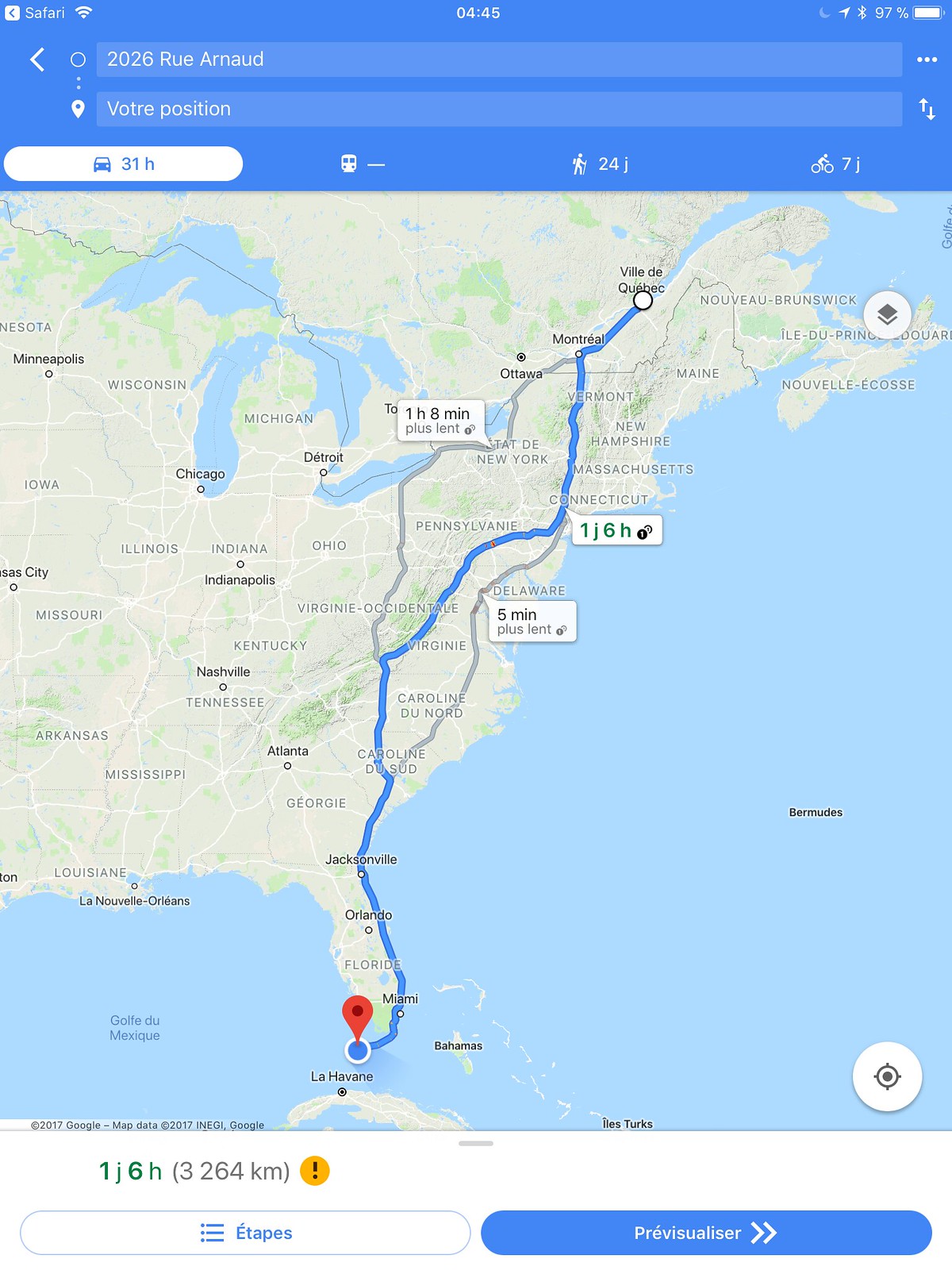A screen capture showing a Google Maps search for directions from a user's current position, indicated as "Votre Position," to 2026 Rue Arnaud, Quebec. The route, entirely displayed in French, calculates a 31-hour car journey covering a distance of 3,264 kilometers to the specified address on Rue Arnaud. The interface exhibits standard map labels and navigation details, all presented in French, reflecting the localized settings of the user's mapping application. The map visually represents the plotted course with highlighted paths and major waypoints between Quebec and the destination address.